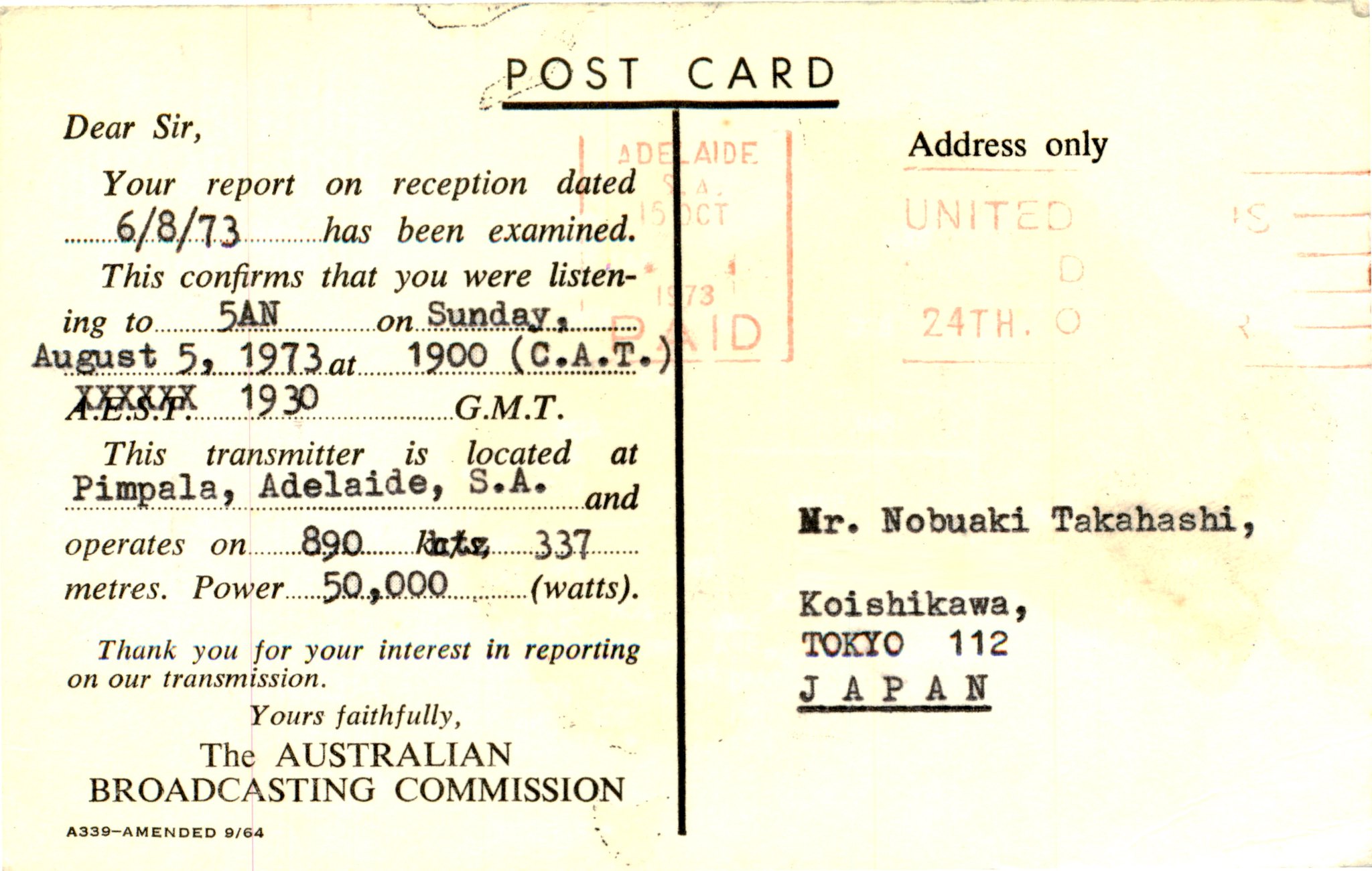This image features a vintage postcard, distinctly aged with a yellowish tint, and worn at the edges. At the top, in bold black text, it reads "Postcard." The left side of the postcard displays a detailed formal letter addressed to "Dear Sir," confirming the receiver's report on reception data dated June 8, 1973. The letter particularly acknowledges the listener was tuned in on Sunday, August 5th, 1973, at 5 a.m. and 1900 C.A.T., 1930 GMT. Notably, the transmitter, identified as operating on 890 kilohertz with a power of 50,000 watts, is located in Pampala, Adelaide, South Australia. The card is signed by the Australian Broadcasting Commission, expressing gratitude for the recipient's interest in the transmission.

To the right, the address field is marked "Address only," prominently featuring the destination address: Mr. Noribaki Takahashi, Koyushiku, Tokyo, Japan, 2012. "Japan" is notably underlined. Multiple red postage stamps from the United States Postal Service, including markings such as “Paid,” “United,” and “24th,” are stamped on this side of the card. The letter text appears to have blank spaces filled in via a typewriter, underscoring its historical value and method of creation.